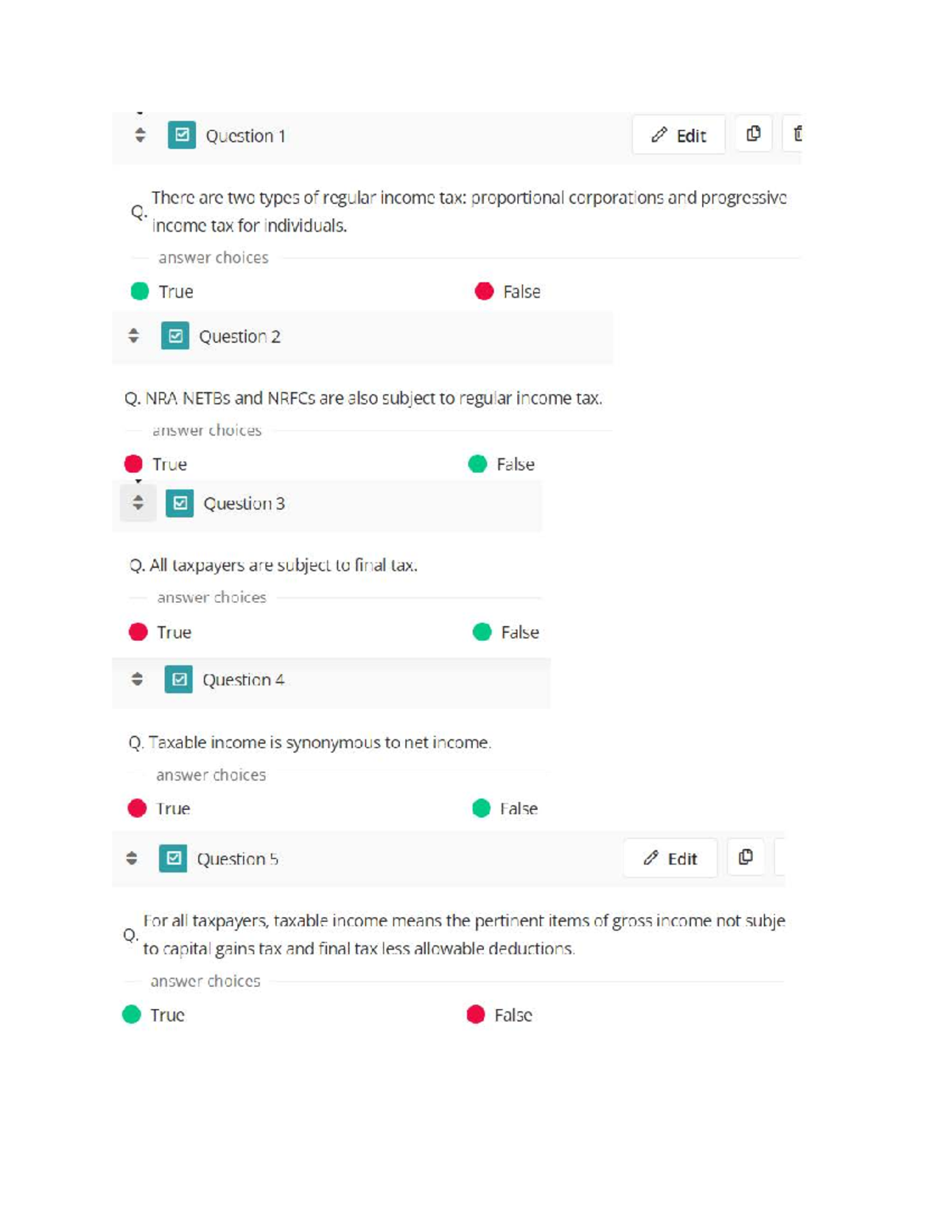This image is a screenshot of an application designed to test the user's knowledge on tax-related statements. The interface presents a series of questions, prompting the user to determine whether each statement is true or false. The first question posed is: "There are two types of regular income tax: proportional corporations and progressive income tax for individuals." Following this, the second question asks whether "NRA and NTBs and NRFCs are also subject to regular income tax." The third question challenges the user with: "All taxpayers are subject to final tax," while the fourth states: "Taxable income is synonymous with net income." The final question in the series reads: "For all taxpayers, taxable income means the pertinent items of gross income not subject to capital gains tax and final tax less allowable deductions." The application also features options to edit or copy the questions, suggesting a customizable and interactive experience for users to engage with the content.